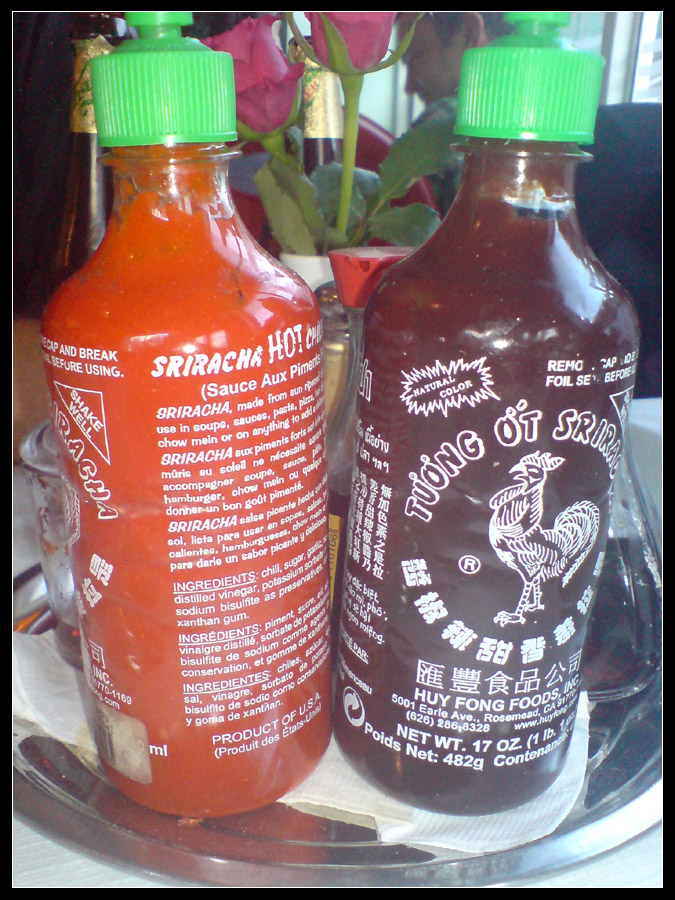This close-up image captures two distinctive bottles of sriracha sauce resting on a silver plate atop a white table. Both plastic bottles are adorned with neon lime green caps and feature the standard sriracha labels, including the iconic white rooster artwork. The bottle on the left contains a bright reddish-orange sauce labeled "Sriracha Hot," while the bottle on the right has a darker brown sauce labeled "Tuong OT Sriracha," with the additional note of it being a natural color. Though the majority of the text on the bottles is not in English, key details such as their weight (17 ounces) and the origin (Hui Fong Foods, Product of USA) are visible.

In the background, a cluster of pink or fuchsia-colored roses emerges from a pot, adding a touch of elegance to the scene. Additionally, a man hovers just above one of the bottles, barely within the frame and appearing to look downwards, possibly engaged in a meal. There are indications of more items on the silver tray, but they are obscured by the prominently placed sriracha bottles. Further back, a couple of champagne bottles can be faintly seen, suggesting a festive or dining setting.